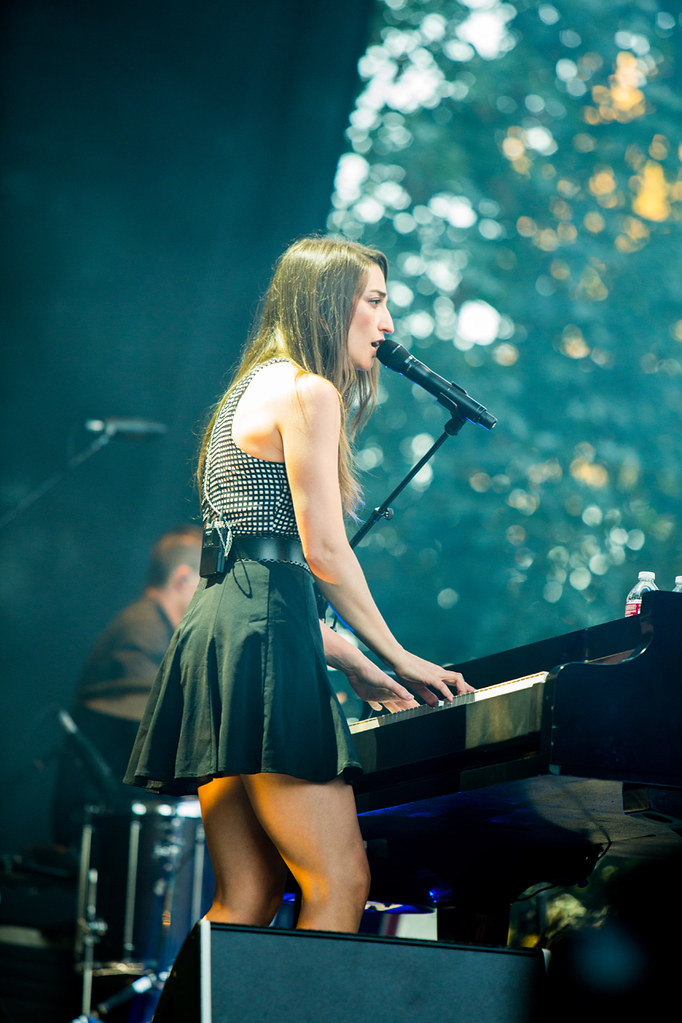In this detailed image, a white female singer with mid-length brunette hair is shown in a back and side profile as she stands at a keyboard with both hands poised to play. She sings into a microphone attached to the keyboard on a stand. Dressed in a short black mini skirt and a white and black top, she also has a battery pack around her waist. The foreground reveals a stage setting with a black background and several shiny silver decorations on the top right. A box, possibly a stage light or speaker, is visible at her feet. To her left, a male figure, depicted only by the back of his head, one ear, and a dark shirt, appears to be playing a bass drum between them.